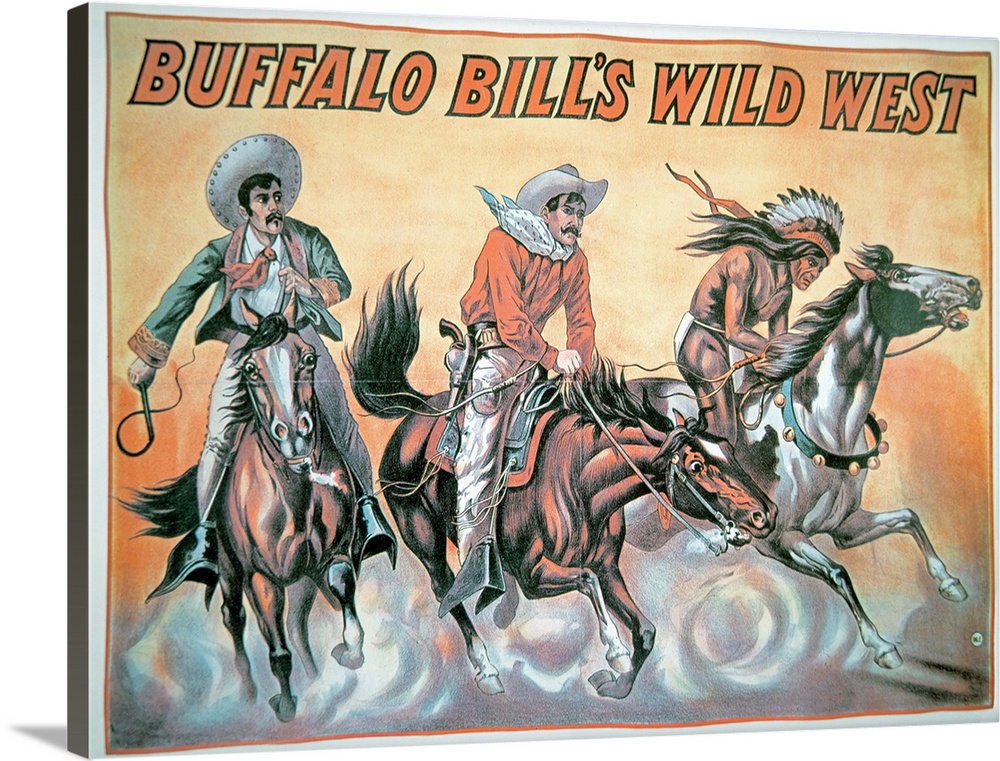This vintage artwork, depicted in a horizontal rectangular frame and photographed at a slight angle, showcases a dynamic scene of three men riding horses against a vivid yellow and orange background. The top of the image prominently features the text "Buffalo Bill's Wild West" in bold orange letters, suggesting it could be an advertisement or a poster from a few years ago.

The central focus of the drawing includes three muscular, young men, each on horseback, charging forward with dust clouds beneath their horses, enhancing the sense of rapid motion. On the left, a Mexican man, identifiable by his sombrero and whip, guides his black horse. In the middle, a classic cowboy clad in a red shirt and white pants, with a gun in a hip holster and a scarf blowing in the wind, rides a powerful black stallion. On the right, a Native American who is wearing a war bonnet and only a loincloth, bursts forth on a Pinto horse, holding a whip.

The entire composition, with its vibrant colors and energetic poses, evokes the wild, adventurous spirit of Buffalo Bill's Wild West show, captured in a detailed and artistic drawing that is both striking and nostalgic.